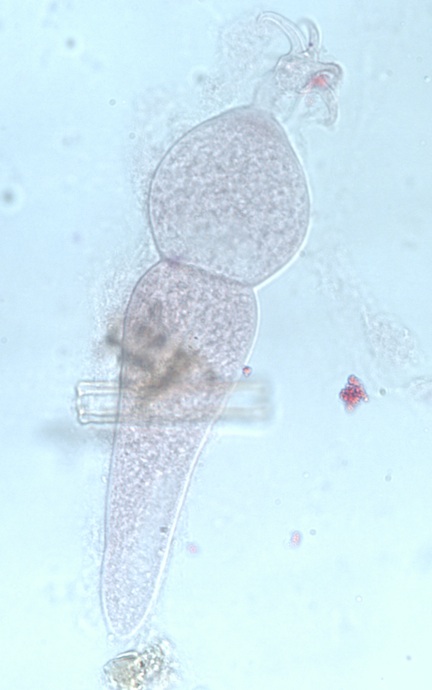This image depicts an extremely magnified microorganism, likely observed through an electron microscope. The organism exhibits a semi-transparent, almost fully translucent body which allows the light-colored background to permeate the entire image. Its structure features a circular, translucent head with hair-like appendages that resemble antennae or tentacles. Below the head, the organism has a slender, elongated thorax, appearing somewhat blobby and gray-white in hue. The background of the image is a light blue or green, reminiscent of a fluid medium such as a petri dish environment. Additionally, there are scattered spots of reddish-purple clusters and other small dots and bubbles in the surrounding area.